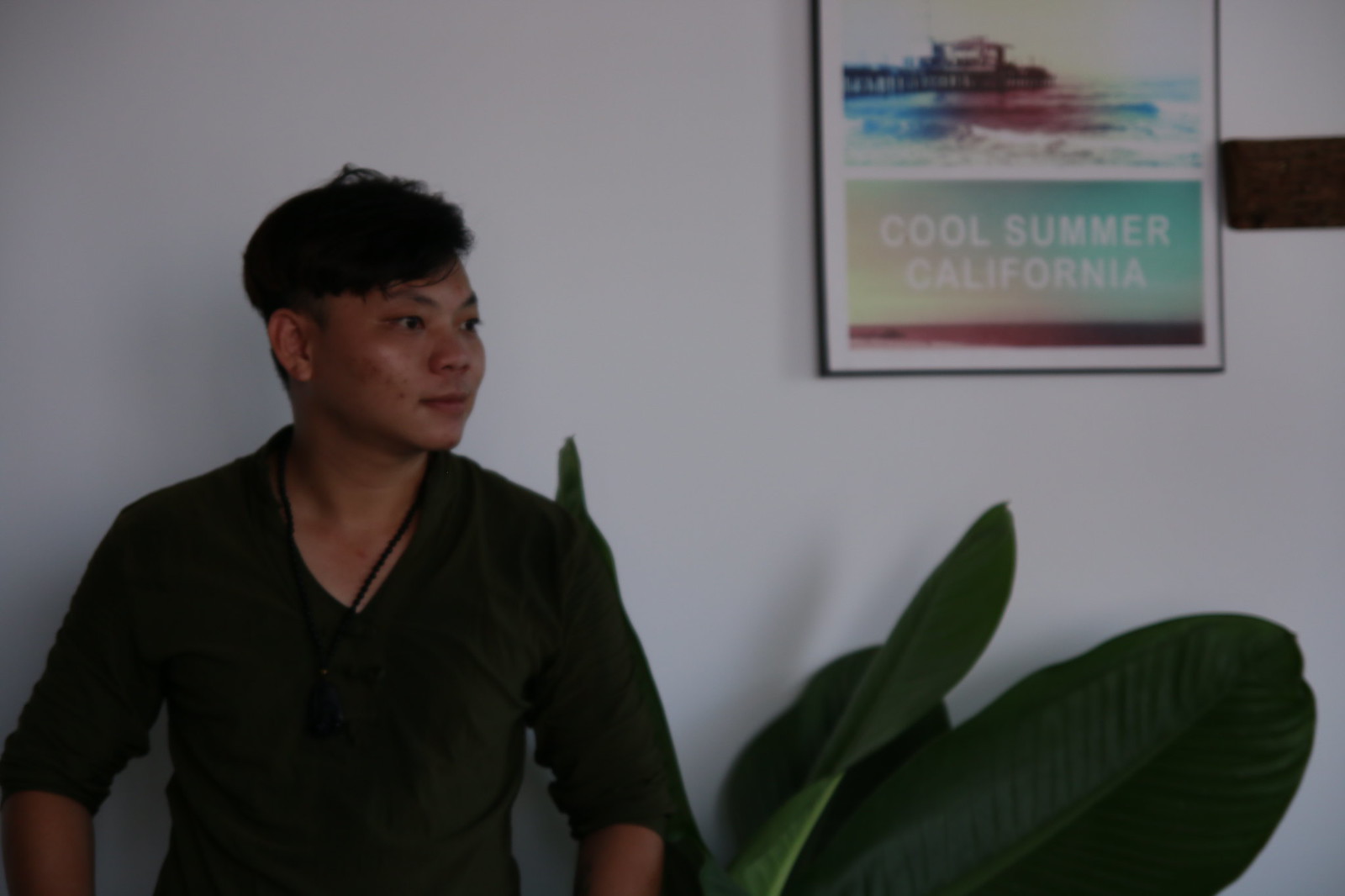This photograph features an Asian male, likely in his late 20s to early 30s, positioned on the left side. He has short hair on the sides and a fuller top, with visible acne scars on his cheek. The man is dressed in a dark V-neck shirt with three-quarter length sleeves and wears a black necklace with a pendant. His gaze is directed towards the right side of the photograph, possibly at another person or object, suggesting a moment of active engagement. The backdrop is a white wall, adding contrast to the darker tones of his attire.

On the right side of the image, partially intruding into the frame, are the large leaves of an indoor plant. Additionally, there is a framed poster on the wall bearing the words "Cool Summer, California," depicting the Santa Monica Pier and ocean waves, hinting at the allure of California. Visible from the man down to slightly above his waist, both he and the plant are cut off at the bottom of the photograph. The image possesses a candid feel, with a slightly out-of-focus and darker quality that implies it might be a still frame from a video.